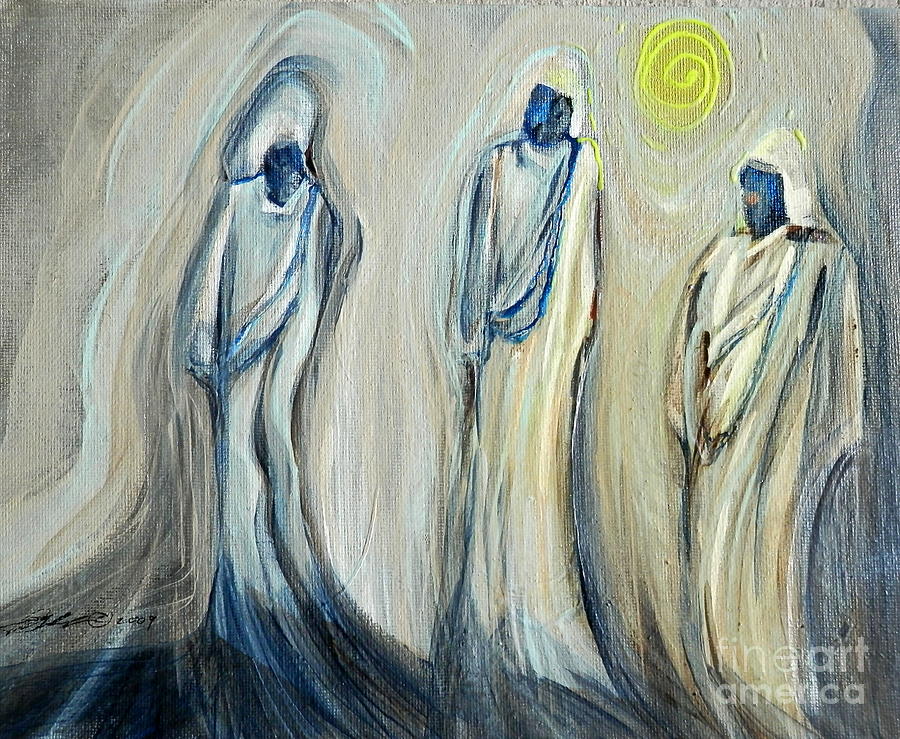The image is a photograph of an abstract painting depicting three humanoid figures clad in white robes, with blue heads devoid of facial features. The painting exudes a sense of religious or spiritual aura, reinforced by their ethereal appearance and the dark blue masses extending from their robes. The background is a cloudy, obscure sky highlighted by a rudimentary, cartoonish yellow sun, represented as a swirl with concentric circles and yellow rays extending outward, casting a glow onto the figures below. The sun is situated towards the top and right side of the canvas, contributing to a powerfully backlit effect on the figures. The painting has a white-grey-cream backdrop and features a semi-transparent watermark in the lower right corner with the Fine Arts America logo. Additionally, a dark signature dated 2009 is visible in the lower left corner, suggesting the artist's identification and the creation date.